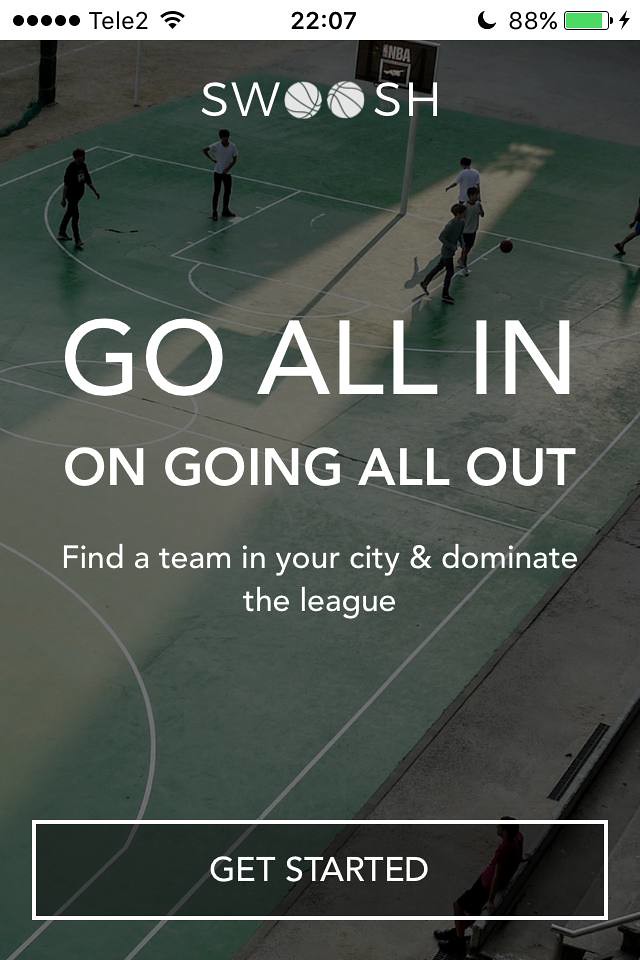The screenshot captures an advertisement on a website, taken from a phone screen. The top of the screen displays typical phone indicators: "Tele2" network, Wi-Fi connection icon, the time "22:07," and an 88% battery with a charging icon. The main ad image below these indicators features a darker-toned image of an outdoor basketball court with five people playing half-court basketball. A ray of sunlight streams down the middle, casting a long shadow from the basketball hoop.

At the top of the ad, the word "Swoosh" is prominently displayed in white letters, with the two 'O's stylized as basketballs. Below this, larger white text reads, "Go all in on going all out. Find a team in your city and dominate the league." At the bottom of the image, a darker button with a white outline contains the text "Get Started." This setup suggests the ad encourages users to join a basketball league locally.